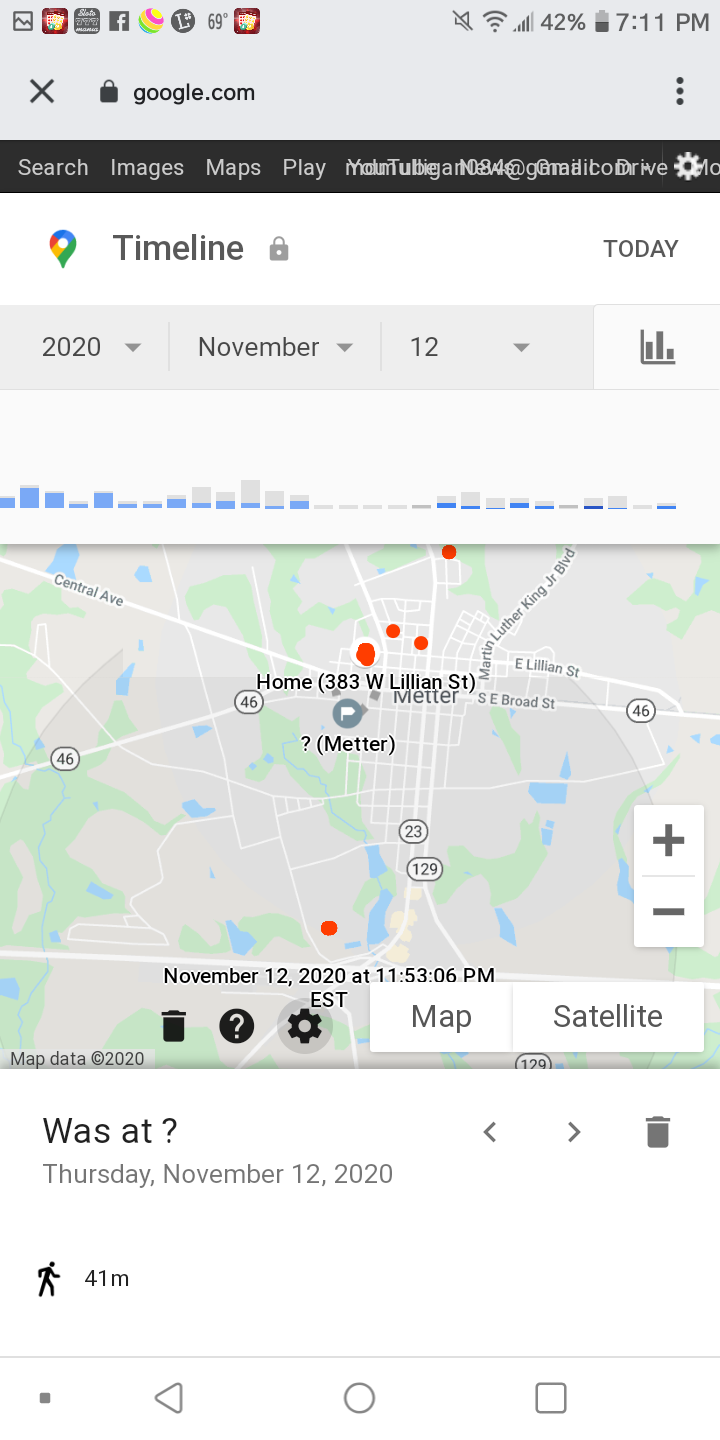Caption: 

On November 12th, 2020, at 11:53:06 p.m. Eastern Time, a Google Maps screenshot displays a series of red dots indicating various locations, alongside a silhouette of a person walking. The map is adorned with various icons, including plus and minus signs, a trash can, a question mark, and settings. The top of the screen shows standard Google services including images, maps, and Google Play. Additionally, the device shows a battery level of 42%. The display features a navigation bar with gray square, triangle, and circle icons, enhancing the detailed interface.